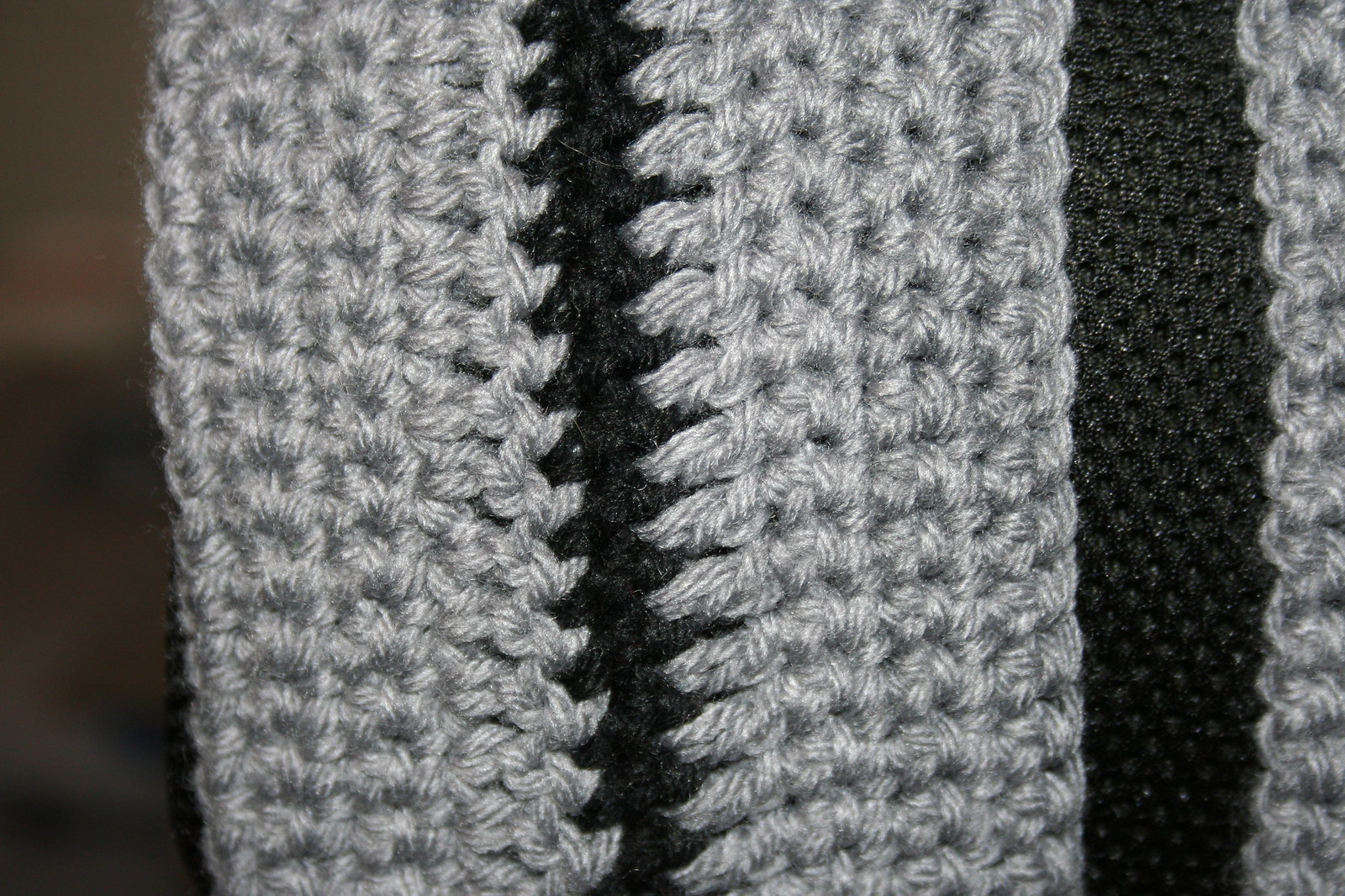This close-up, black-and-white photograph showcases a hand-knitted or crocheted material, possibly a sweater, blanket, or scarf. Dominating the center and right side of the image, the fabric is meticulously detailed with various decorative stitching patterns. The yarn is grayscale, displaying hues from stark black to shades of gray. The knitting features several sections: on the far right, a white section transitions into a thicker, black segment interspersed with small holes. This is followed by a broader white section and then a very thin black strip with outward lines, culminating in a thick swatch of white yarn on the far left. Despite the lack of a date, location, person, timestamp, or text, the photograph captures the warmth and intricate design of the fabric, making it a compelling study of textured craft.